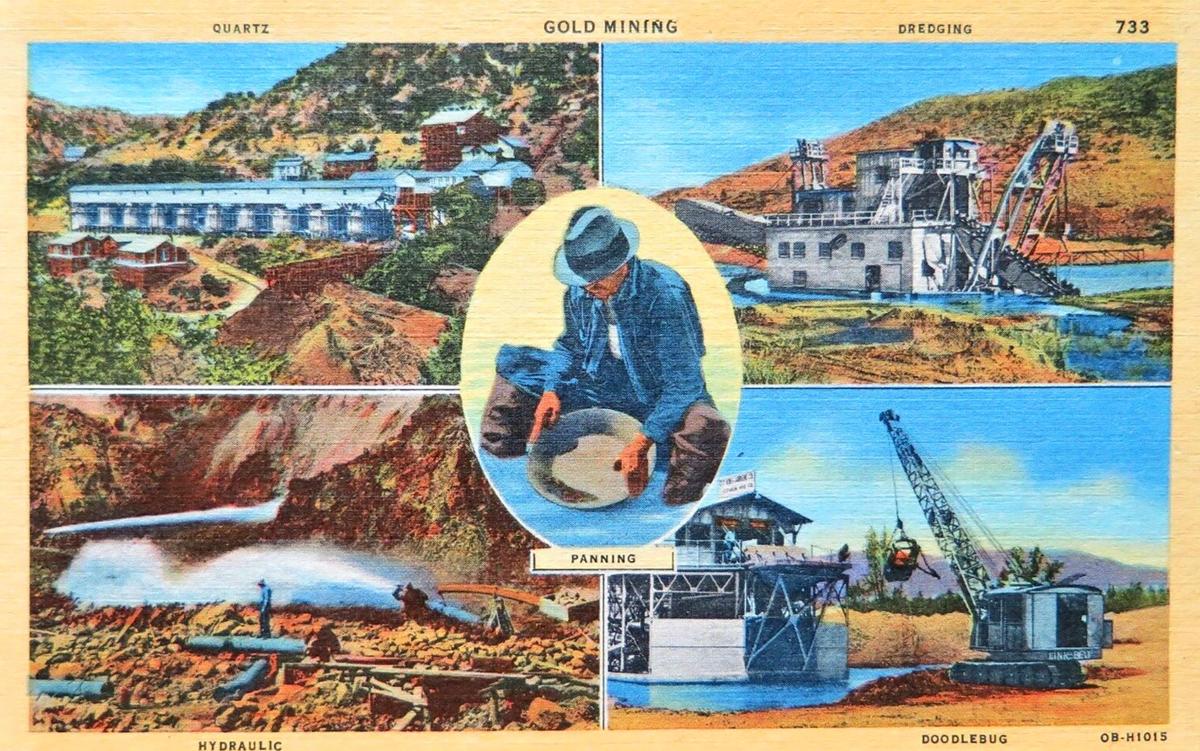This detailed illustration depicts various historical gold mining methods, arranged in a structured layout with a clear tan background. At the top left corner, there's a detailed drawing of a large factory or mine-like building, with the word "quartz" written above it in black. Adjacent to it in the top right corner is a depiction of a square, white riverboat equipped with extensive machinery, labeled "dredging." In the bottom left, a miner operates a large pipe, directing high-pressured water against a mountainside to dislodge dirt, illustrating the "hydraulic" technique.

Centered within the image is an oval scene of a miner clad in a blue jacket and hat, intently looking down into a pan, engaged in the process of gold panning. Surrounding this central figure are four rectangular illustrations, each showcasing different aspects and machinery associated with gold mining, all set against a rugged backdrop of mountains and debris. The imagery collectively captures the multifaceted and labor-intensive nature of historical gold mining practices.